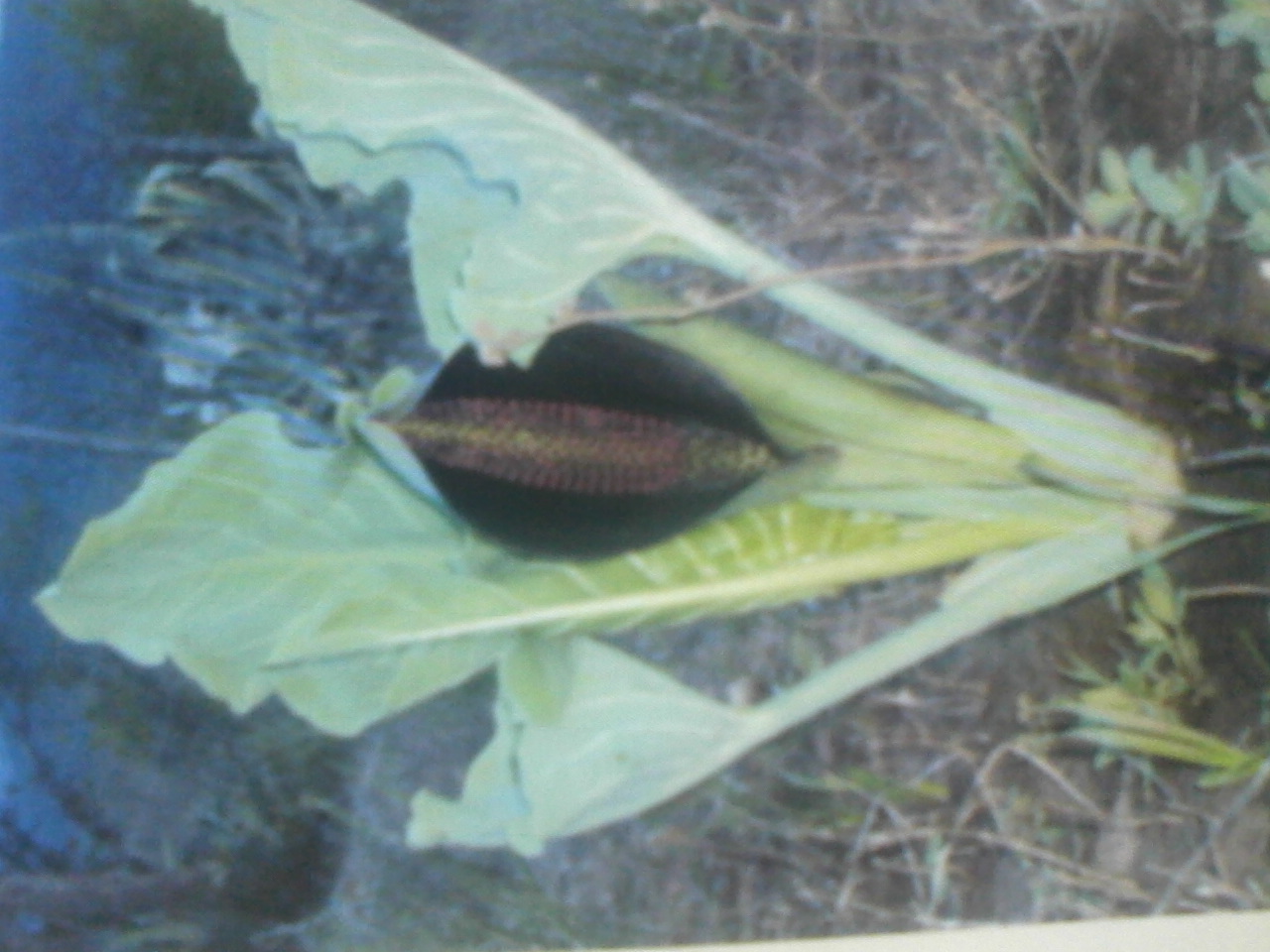This slightly blurry photo, taken at an odd, tilted angle of about 90 degrees to the left, showcases a distinctive plant with an intriguing structure. The plant appears to be growing outdoors amidst dirt, soil, grass, and scattered twigs, with trees and a dark blue sky suggesting it was captured early in the morning or late in the evening under ambiguous lighting conditions. The plant is characterized by large, floppy green leaves with white veins that resemble those of a cabbage. At its center, there is a peculiar, tubular structure with deep brown, lighter-striped markings that evoke the appearance of a corn cob, adding to the plant's enigmatic nature. Despite the challenging angle and blur, the image vividly portrays an unusual vegetable sprouting amidst a natural, rustic setting.